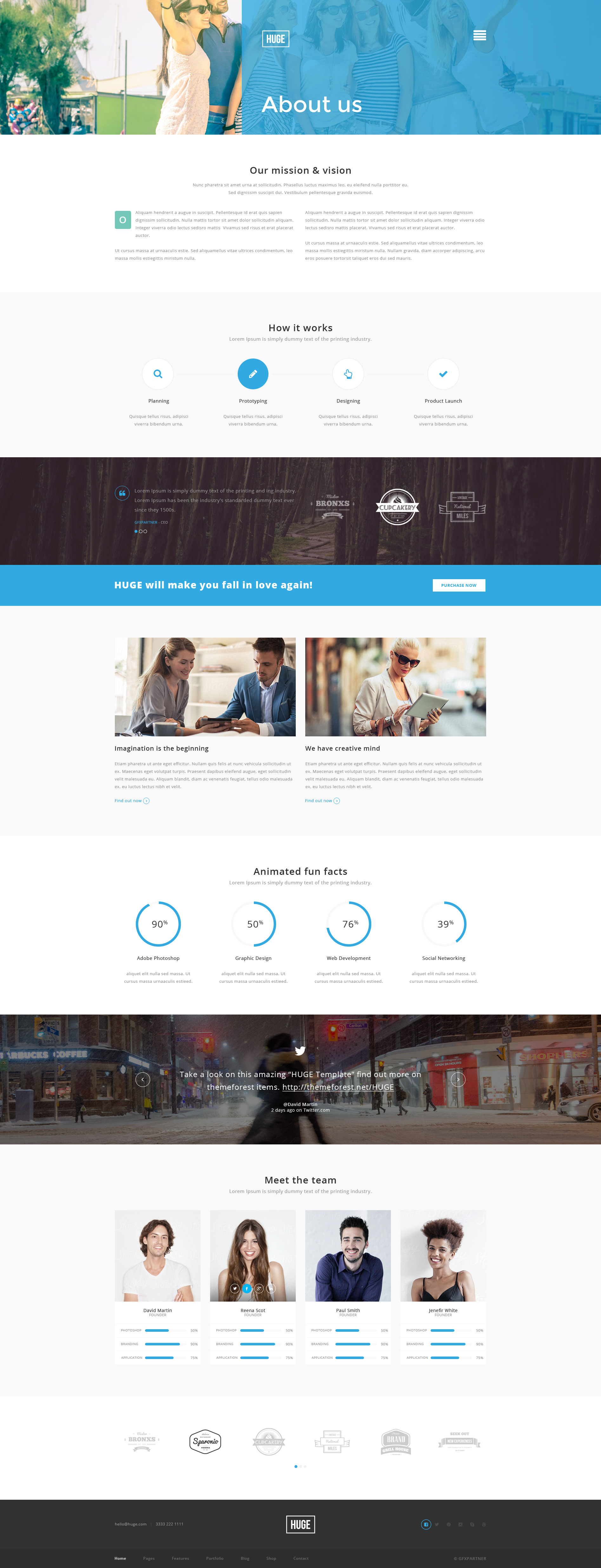This is a detailed screenshot of an "About Us" page from a company's website. The image is tall and contains multiple sections, organized to provide comprehensive information about the company. Notably, the screenshot captures only the content of the page without any browser UI elements.

### Header Section
- **Left Side**: Features a photo of a man and a woman in an outdoor setting with a greenery backdrop.
- **Right Side**: This sub-section occupies 60% of the header area. It showcases an image of five women overlaid with a blue tint. Superimposed on this image is the text "About Us" in white.

### Central Content
- **Main Heading**: Centrally aligned, bold black text (indecipherable due to the small size).
- **Subheading & Paragraph**: Located directly below the main heading with centrally aligned content.
- **Split Paragraph Sections**: Two columns of paragraph text, left and right-aligned, both set on a white background but too small to read.

### Icons Preview Section
- **Background**: Light gray.
- **Content**: Features four icons, each with subheading text and detailed descriptions below them.

### Photo Overlay Section
- **Background**: Dark overlay on a photo, making it difficult to see details.
- **Text and Icons**: Small white text alongside logos/icons, challenging to read.

### Blue Bar Section
- **Background**: Blue.
- **Content**: White text stretched across the bar with a white button on the right end.

### Information Boxes Section
- **Layout**: Two boxes, left and right.
- **Left Box**: 
  - **Image**: Shows a woman and a man seated, concentrating on an item on a table.
  - **Text**: A heading followed by a paragraph beneath the image.
- **Right Box**: 
  - **Image**: Depicts a woman using a tablet.
  - **Text**: Black bold heading with a paragraph below.

### Percent Circles Section
- **Background**: White.
- **Content**: Circles displaying percentages, labeled with headings and descriptions.

### Quote Overlay Section
- **Background**: Dark overlay on an image.
- **Text**: White text in the center, possibly a quote.

### Meet the Team Section
- **Title**: "Meet the Team" at the top.
- **Images of Team Members**:
  - **Individuals**: Two men and two women.
  - **Details**: Text under each person with blue bars below.
  
### Company Logos Section
- **Content**: Logos of various companies presumed to be clients or partners.

### Footer Section
- **Background**: Black.
- **Content**: White text and icons, which are, however, too small to read.

This structured overview aims to provide a comprehensive understanding of the visual layout and the content distribution across the "About Us" page, emphasizing the organizational flow and the visual elements present.